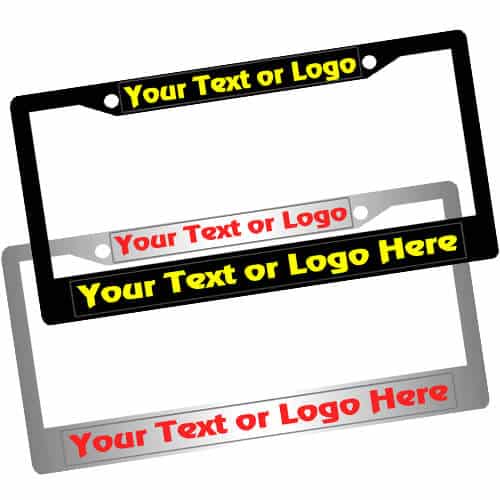This image features a product photograph showcasing two customizable license plate frames, set against a blank white background. The frames are designed to enable personalized text or logos. The black frame, positioned on top and slightly overlapping the silver frame, displays bold, neon yellow text that reads "your text or logo" at the top and "your text or logo here" at the bottom. Both pieces of text are flanked by two white circles, likely screw holes for mounting. The silver or metallic gray frame beneath it features the same text placement and white screw holes, but the text color is a muted red. The frames are displayed in a way that highlights their customization and design options, with the black frame resting slightly above and to the right of the silver frame.